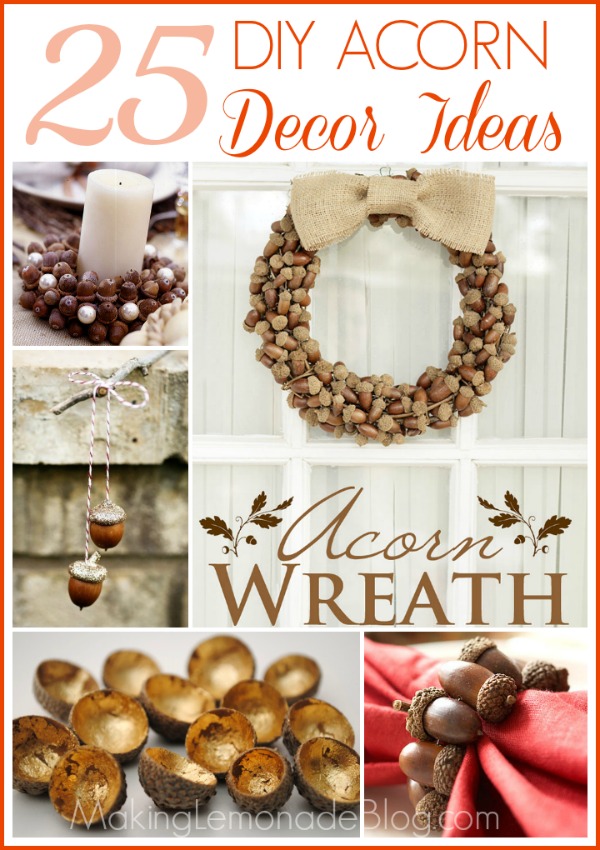This vertically-oriented graphic, likely designed for social media or a blog, features a red outline and white background with multiple detailed photographs of acorn decorations. At the top, the title "25 DIY Acorn Decor Ideas" is prominently displayed in red font. Centered in brown text is the label "Acorn Wreath," highlighting the main design element. At the bottom, a subtle white watermark reads "makinglemonadeblog.com."

The graphic includes several realistic, edited-together photographs showcasing various acorn decor ideas. The upper section features a festive candle centerpiece surrounded by acorns. Just below, acorns are creatively tied to a red and white string, hanging from a twig. A central panel highlights an elegant acorn wreath adorned with a large beige bow, accompanied by the caption "Acorn Wreath." Another image presents acorns halved and painted gold, demonstrating a sophisticated craft idea. Finally, at the bottom right, acorns are strung together to form a charming napkin holder, perfect for rustic table settings. This comprehensive visual guide offers multiple inspiring ways to incorporate acorns into your home decor.